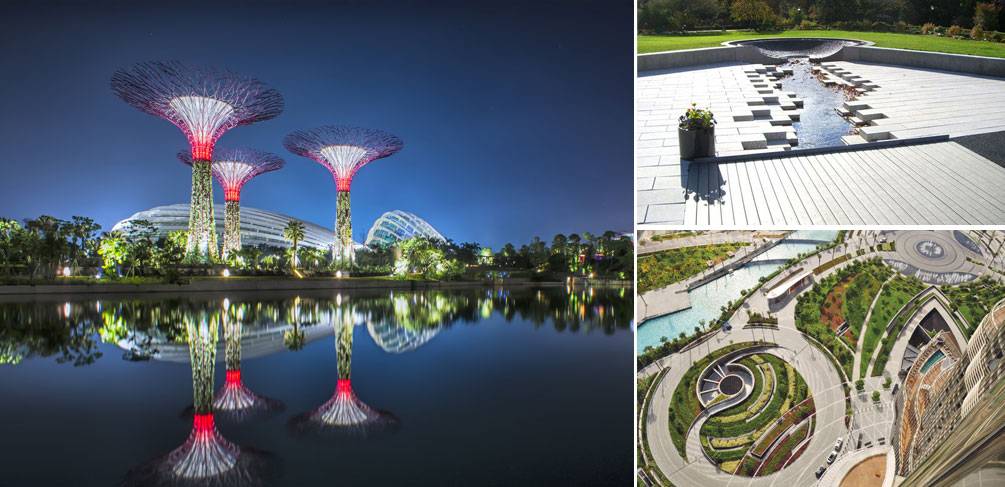The collage features three compelling images with the left-side image showcasing an iconic and futuristic building reminiscent of the Sydney Opera House, bathed in the serene hues of a nighttime scene. The structure, resembling an oval with a smaller dome behind it, sits beside a smooth, reflective body of blue water. In front of the building, three towering LED light installations dominate the scene, their bases wide and green, narrowing as they ascend and morph into vibrant pink, purple, then an extended fanned-out top. The light structures are mirrored perfectly on the water, enhancing their mesmerizing display.

The upper right image captures a picturesque stone or brick patio area with a deliberate, design-heavy water feature running through its center from a bowl-like sculpture. The scene, rich with lush greenery including grass, trees, and plants, is a tranquil, intimate part of a garden or park.

The lower right image offers an aerial perspective, looking down on a sophisticated landscape. The vista encompasses a circular pathway guiding through an organized garden layout, a flowing river, and tranquil walking paths. Buildings punctuate the greenery, emphasizing a harmonious blend of urban and natural elements in this seemingly futuristic and meticulously planned space.